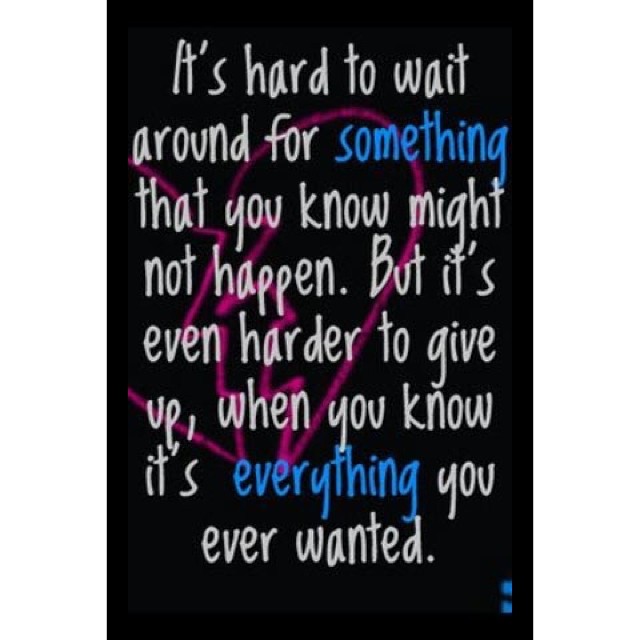The image features a poignant quote overlaying a visually striking background on what seems to be a social media graphic. The background is entirely black, providing a stark contrast to the pink broken heart in the center. The heart, possibly representing emotional pain or loss, is rendered in a slanted style, with a humorous, slanted font used for the overlaid text. The quote reads, "It's hard to wait around for something that you know might not happen. But it's even harder to give up when you know it's everything you ever wanted." Notably, the words "something" and "everything" are highlighted in blue, while the rest of the text is in white, emphasizing the emotional weight of those words. In the bottom right corner, two blue dots are arranged vertically, adding a minimalistic design element. The entire image is in portrait orientation, typical of a phone screen capture.